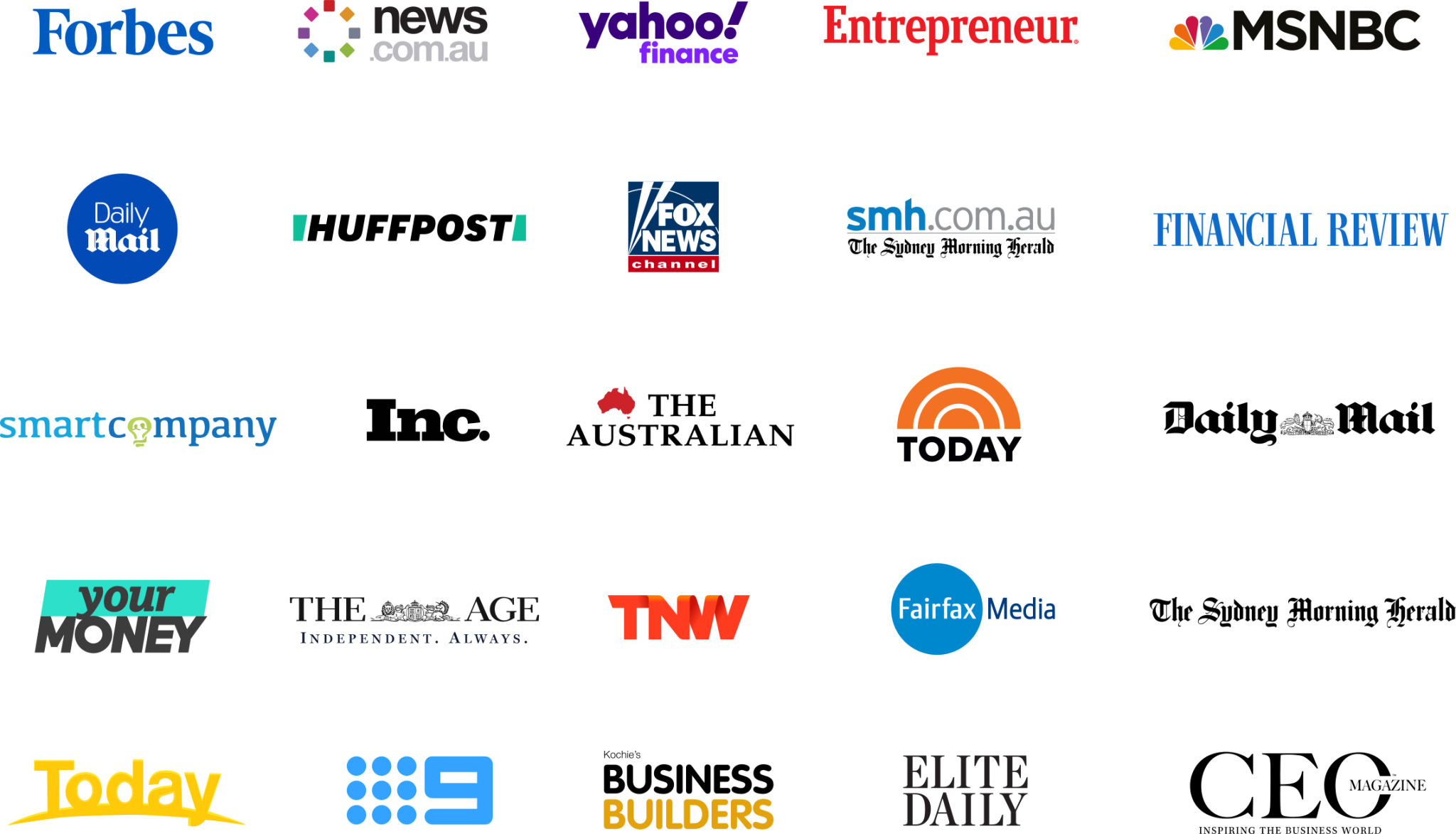This image showcases the names and icons of various media companies arranged in a grid format consisting of five rows and five columns. Here is a detailed breakdown of the arrangement and description of each icon:

### **Top Row:**
1. **Forbes** - The word "Forbes" written in blue lettering on a white background.
2. **news.com.au** - Features multiple small squares in a circular arrangement, displaying various colors like a rainbow.
3. **Yahoo Finance** - "Yahoo Finance" written in purple on a white background.
4. **Entrepreneur** - The word "Entrepreneur" written in red on a white background.
5. **MSNBC** - Displays the NBC Peacock logo, with "MSNBC" written in black.

### **Second Row:**
6. **Daily Mail** - A blue circle with "Daily Mail" written in white lettering.
7. **HuffPost** - (Description not provided in the original text, but typically green and white)
8. **Fox News Channel** - Features the logo with "Fox" in bold letters and "News Channel" underneath.
9. **smh.com.au (Sydney Morning Herald)** - (Description not provided in the original text, typically black and white)
10. **Financial Review** - (Description not provided in the original text, typically blue and white)

### **Third Row:**
11. **SmartCompany** - (Description not provided in the original text)
12. **Inc.** - Typically written in bold black font on a white background.
13. **The Australian** - (Description not provided in the original text)
14. **Today** - (Description not provided in the original text)
15. **Daily Mail** - Repeating icon of the blue circle with "Daily Mail" in white lettering.

### **Fourth Row:**
16. **Your Money** - (Description not provided in the original text)
17. **The Age** - (Description not provided in the original text)
18. **Independent Always** - (Presumably referring to "Independent" with a tagline "Always". Description not detailed)
19. **TNW (The Next Web)** - (Description not provided but their logo is typically in orange and white)
20. **Fairfax Media** - (Description not provided in the original text)

### **Fifth Row:**
21. **Sydney Morning Herald** - (Repeated entry from the second row)
22. **Today (Second entry)** - (Repeated entry from the third row)
23. **Nine** - (Description not provided, but typically blue and black with the number nine in pixels)
24. **Cochise The Business Builders** - (Description not detailed)
25. **Elite Daily** - (Description not provided in the original text, typically black and white) 
26. **CEO Magazine: Inspiring the Business World** - Displaying "CEO Magazine" with a tagline "Inspiring the Business World" (Description not detailed)

This comprehensive description aligns the names and icons in a systematic way, allowing for easy identification and visualization of each media company represented in the image.